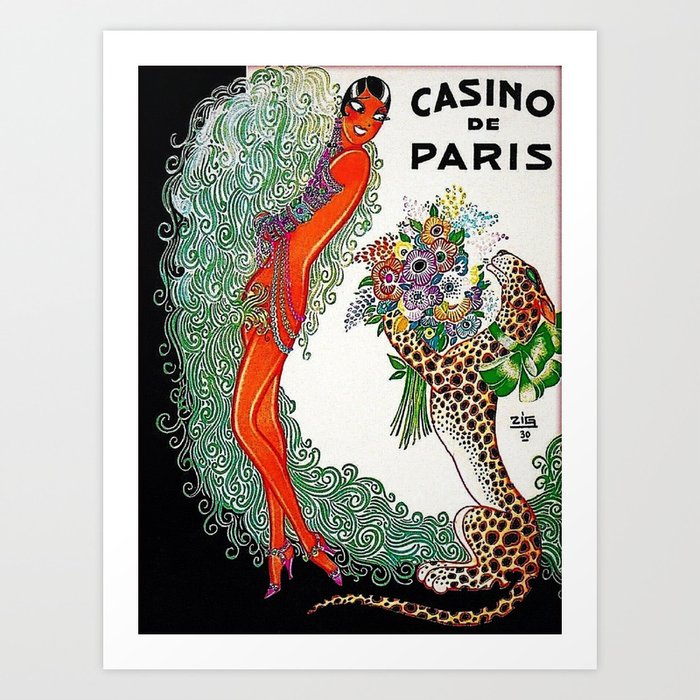The poster titled "Casino de Paris" features a striking illustration against a neutral light blue background with a thick white border. The title is written in black, all capital letters with "de" appearing smaller, and the word "Casino" is artistically curved. At the center of the image, a woman reminiscent of the 1920s style is prominently displayed. She has red skin, short black hair, and is adorned with intricate green swirl patterns on her arms, along with substantial jewelry. She appears to be wearing or draped in a luxurious, feathery gown. This elegant figure gazes downwards at a vibrant orange leopard with black spots, which stands on its hind legs. The leopard, wearing a green belt, presents the woman with a diverse bouquet of colorful flowers, including purple, yellow, and orange hues. The vibrant poster is awash with lively colors, featuring bold oranges, greens, purples, and yellows, enhancing its eye-catching appeal.